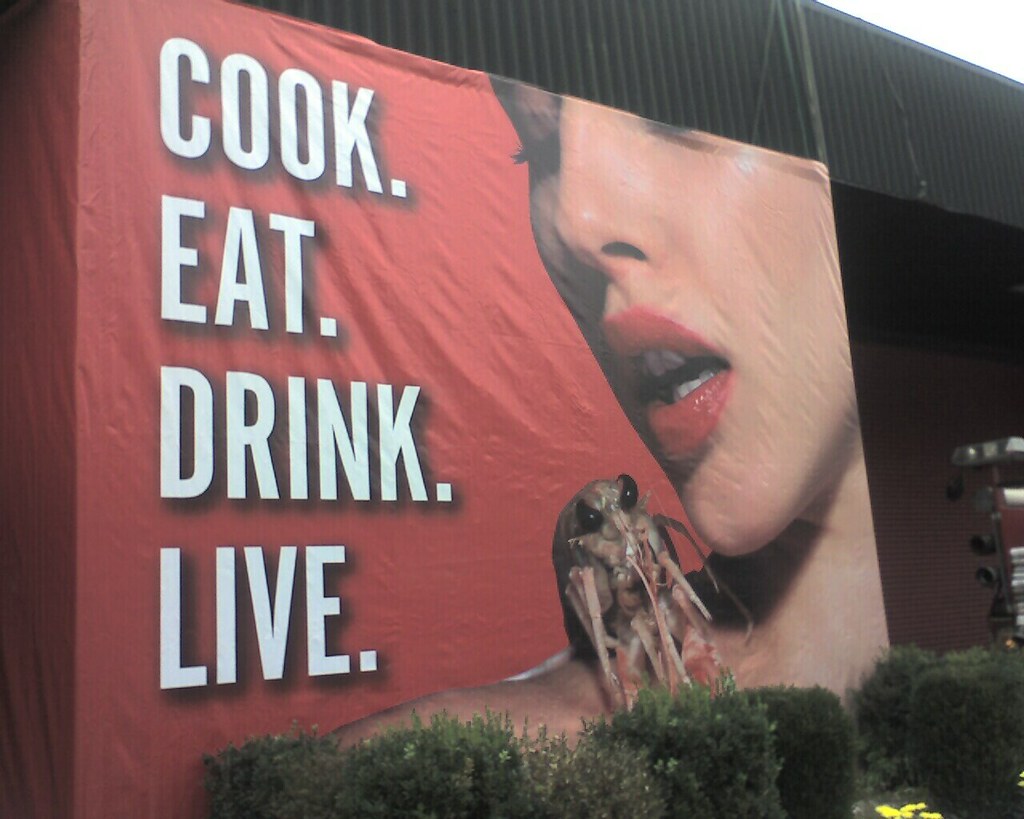In this outdoor photograph, a vibrant sign commands attention. Positioned against a building, the sign is surrounded by a brick wall on the right and a dark-colored exterior wall above it. The clear, light sky peeks through in the top right corner, adding an airy backdrop to the scene. The sign itself is primarily red with bold white lettering, presenting the words "Cook," "Eat," "Drink," and "Live" on separate lines.

Adjacent to the sign on the right, a striking image of a woman's face extends to include her neck and right shoulder. Her eyes are closed, and lips painted a vivid red, slightly parted, giving her an enigmatic expression. Perched delicately on her shoulder is a small shrimp or crawfish, adding an unusual yet intriguing element to the image. Beneath the sign, lush green bushes add a touch of natural vibrancy to the scene.